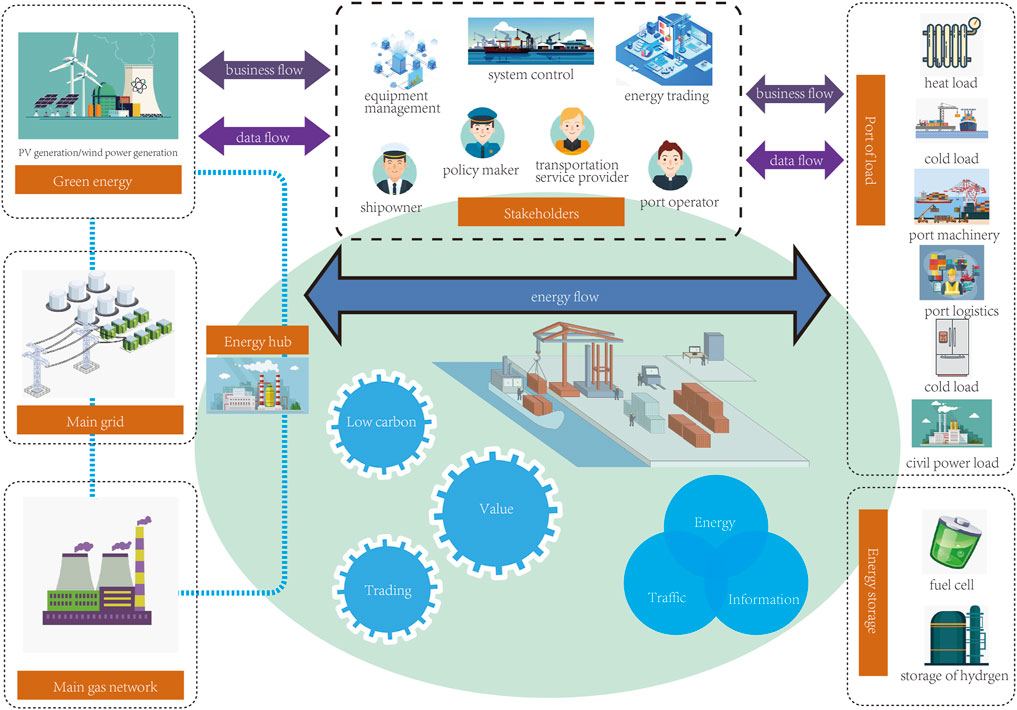This is an animated image of an energy flow chart that intricately details the various stages and stakeholders involved in green energy production and distribution. On the left, there are several 3D illustrations, including a nuclear power plant and windmills, labeled as "green energy". Below this, we see the "main grid" depicted with white cylindrical structures and green cubes, and further down is the "main gas network" illustrated with smokestacks. Above these, purple dual arrows labeled "business flow" and "data flow" indicate the movement of information and services.

In the center of the chart, a long blue double arrow represents the "energy flow". Adjacent to this central section, we find the primary stakeholders: ship owners, policymakers, transportation service providers, and port operators. This segment emphasizes the collaborative effort required to manage energy transfers.

At the bottom, within a green circle with blue spheres, it reads "low carbon value and trading" and "energy traffic information," signifying environmental and informational components of the process.

On the far right, various loads and functions are illustrated, including "heat load," "cold load," "port machinery," "port logistics," and "civil power load." This section is also marked by "business flow" and "data flow" arrows, reiterating the continuous exchange of data and business activities.

Each step of this process is represented by distinct animated avatars, showcasing the involvement of different departments and stakeholders in the energy production and flow system. This comprehensive and visually engaging diagram could serve as an educational tool in presentations or textbooks to explain energy transfer and management.